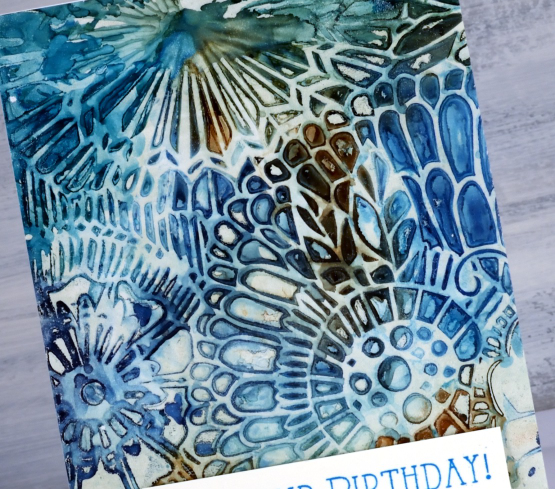This angled view of a watercolor painting captures an abstract blend of shapes and colors, reminiscent of stained glass due to the way the hues mix and radiate. Dominated by various shades of blue with touches of brown, the artwork features an array of indistinct forms, including circles and radial patterns that resemble snowflakes, gears, and flower petals. These elements create a mosaic-like effect, with shapes that are comparable to fingernails and cylinders interspersed throughout. The painting rests on a gray wooden table, and at the bottom center-right of the photo, a portion of a white banner with the blue-lettered capitalized words "HAPPY BIRTHDAY!" can be seen, adding a celebratory context to the scene.